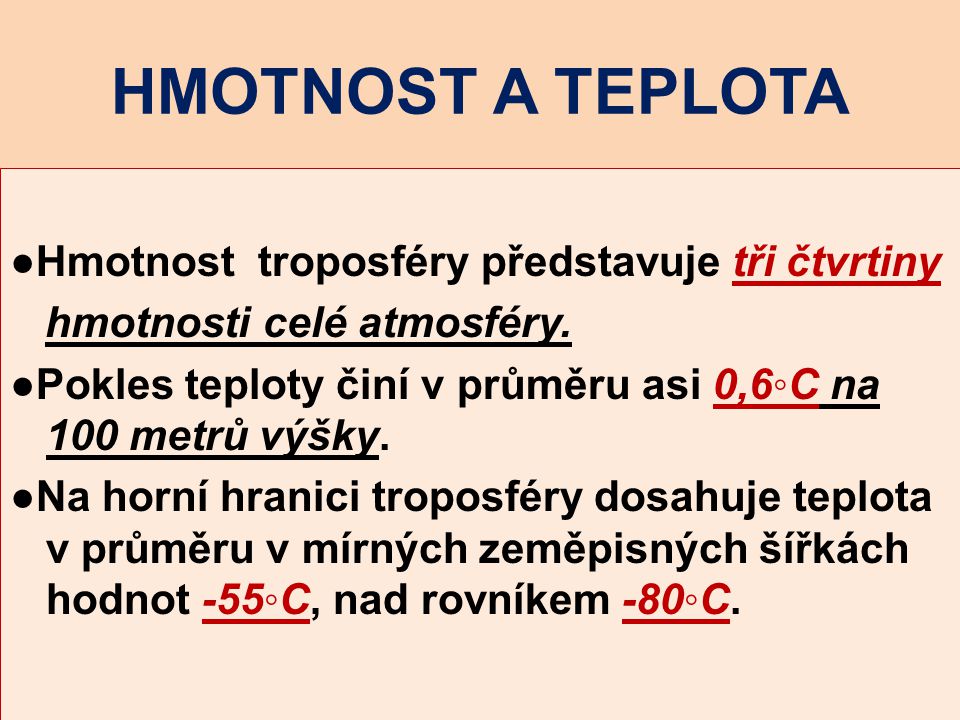The image depicts a sign composed of text in a foreign language. The sign has a predominantly peach-colored background with a slightly darker peach header at the top. In blue, all-caps font, the header reads: H M O T N O S T A T E P L O T A. 

Beneath this header, the background shifts to a lighter pink tone, and the content is organized into three bullet points, each in black text:

1. H M O T N O S T T R O P P O S F E R Y P R E D S T A R U R S T R Y S T R I V N Y H I M N O S T Y S L A T M O S F E R Y
2. P O L K S T E P L O V Y S I N N Y V Y P R U M L U S I Z E R O C O M M A S S I X D E G R E E S C N O W O N H U N D R O O D M E T R O O W I S K Y
3. N A H O R N Y H I R A N S Y T R O P O S F E R Y D O S A H U T A P L O T A V Y P R U M L U V Y M R N I S H Z M S T R I M F I S T S H A K A S H H A T N O T N E G A T I V T H I F T Y F I T D E G R E E S C N O W O N H U N D R O O D N O W I K I M N E G A T I V T H I F T Y T D E G R E E S C.

Notable highlighted values include "0.6 degrees Celsius," "negative 55 degrees Celsius," and "negative 80 degrees Celsius," indicating temperature readings. Some accent marks appear over certain letters, but further specifics of the language remain unclear.